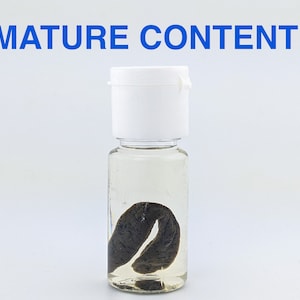The image depicts a small clear bottle with a white cap, positioned against a solid white background. The bottle appears to be filled with a clear, slightly yellowish liquid, suggesting preservation fluid such as formaldehyde. Suspended within the liquid is a dark, shriveled object, curled into a U-shape, and its exact nature is unclear. The cap of the bottle is almost as tall as the bottle itself and is designed like the top of a squeeze bottle. At the very top of the image, in capitalized blue letters resembling an aerial font, the words "MATURE CONTENT" are prominently displayed. The image is brightly lit, ensuring that all details are clear and visible.